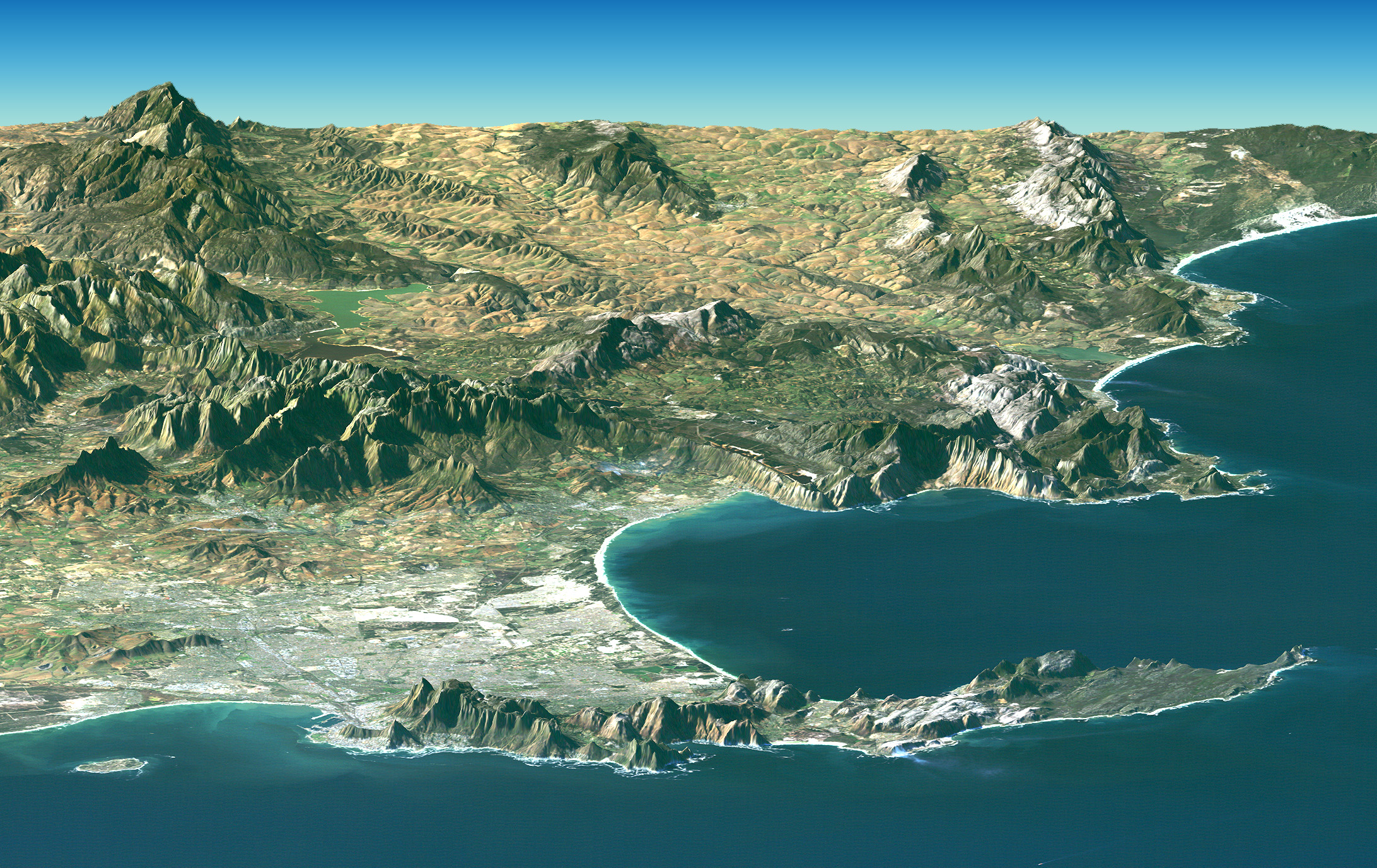This aerial photograph captures a stunning and diverse coastal landscape, characterized by its dark blue waters and curving coastline. In the lower part of the image, a small peninsula, resembling a dragon's mouth, extends into the sea, flanked by rugged cliffs. Another smaller, mountainous peninsula is situated just above it. The right side of the image mostly follows the irregular, curvaceous shoreline, whereas the left side is dominated by imposing mountains and rocky formations in shades of gray and brown. The photograph, taken from an elevated viewpoint, probably an airplane, showcases various terrains: from snow-capped peaks to desert-like, brown expanses and green landscapes. The horizon is visible at the very top, with a clear blue sky occupying the upper 20% of this horizontally oriented, postcard-like image. Small lakes nestled in the valleys and a developed area near the coast add further layers of detail to this vibrant and intricate scene.